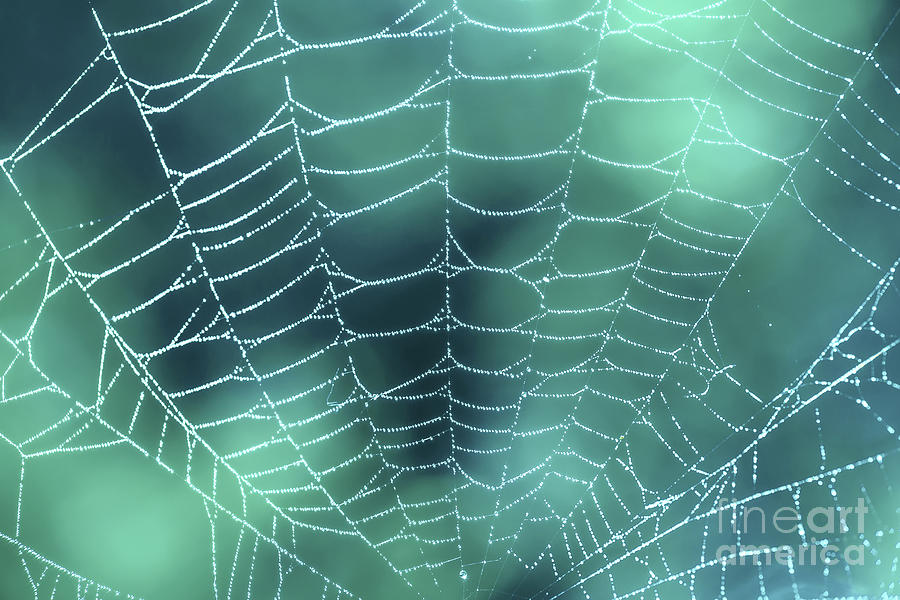This image captures the intricate beauty of a dewy, silvery spiderweb set against a backdrop of varying shades of light and deep green. Illuminated from the top, the web shines almost like it's made of tiny diamonds, giving it an ethereal, almost otherworldly appearance. It features a symmetrical pattern, though there's a notable tear in the bottom left corner. The web arcs gracefully from the bottom, with some strands appearing taut while others have slack or are even broken, adding to its natural charm. Moisture glistens at the center, enhancing its delicate structure. In the bottom right-hand corner, there's a watermark reading "Fine Art America." This might be a poster representing the high-quality artwork offered by the brand, showcasing the spiderweb as a fine example of nature’s artistry.